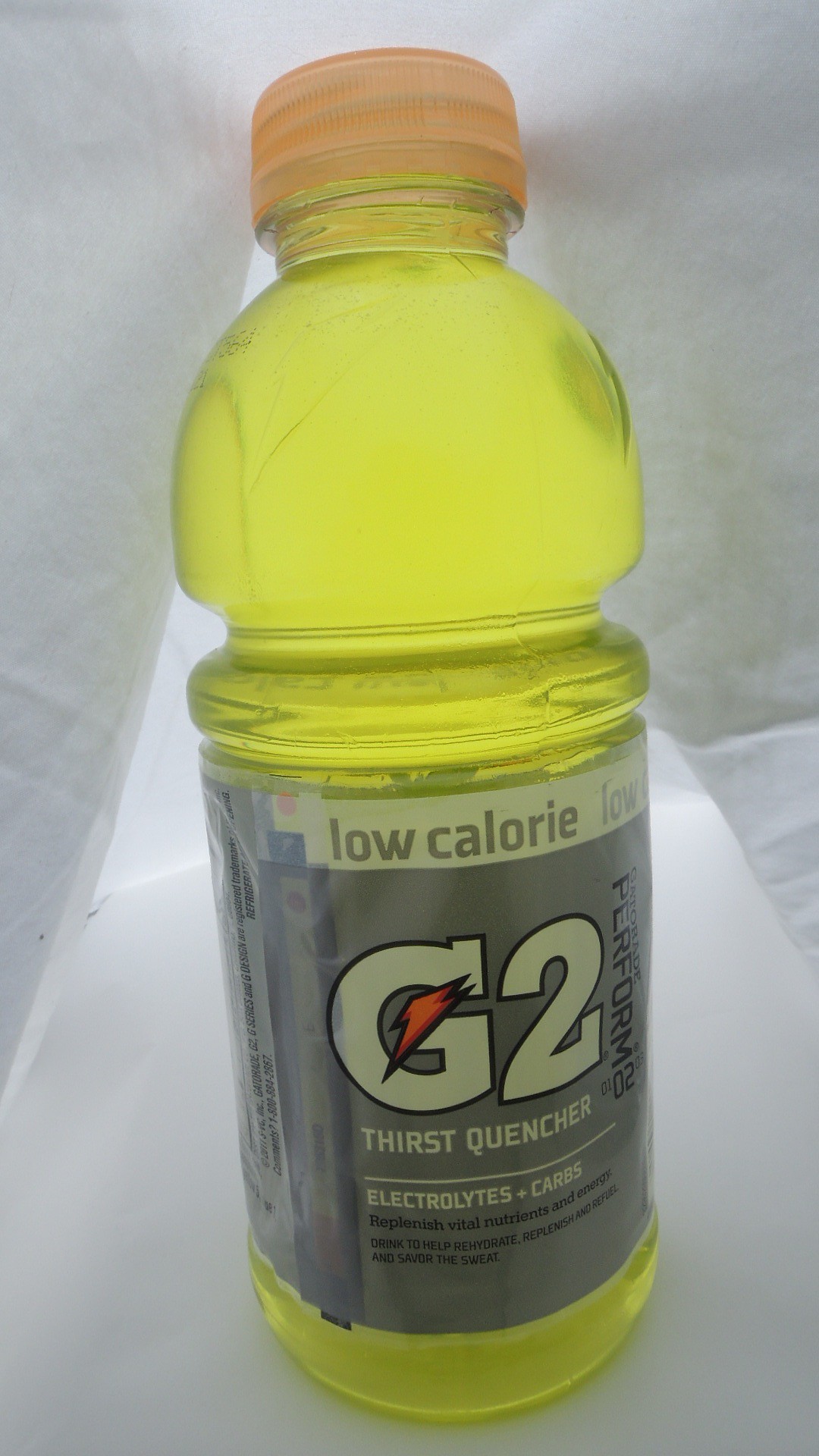This detailed photo showcases a Gatorade G2 bottle, branded as a low-calorie, lemon-lime flavored thirst quencher. The bottle has a distinctive yellow-green color with an orange cap and is set against a white background on a white surface, accompanied by crumpled white paper. The label is predominantly white and gray, with "low calorie" printed on the upper part, followed by "G2" in gray with an orange lightning bolt through the "G". Below this, it states "thirst quencher," and underneath, it mentions "electrolytes + carbs". Additional text indicates it helps replenish vital nutrients, although some of the smaller print is not fully legible. Vertically on the right side of the label, the word "perform" is visible. The image emphasizes the essential details and color contrasts, including the orange cap and black outlines, capturing the essence of this energy-replenishing drink.